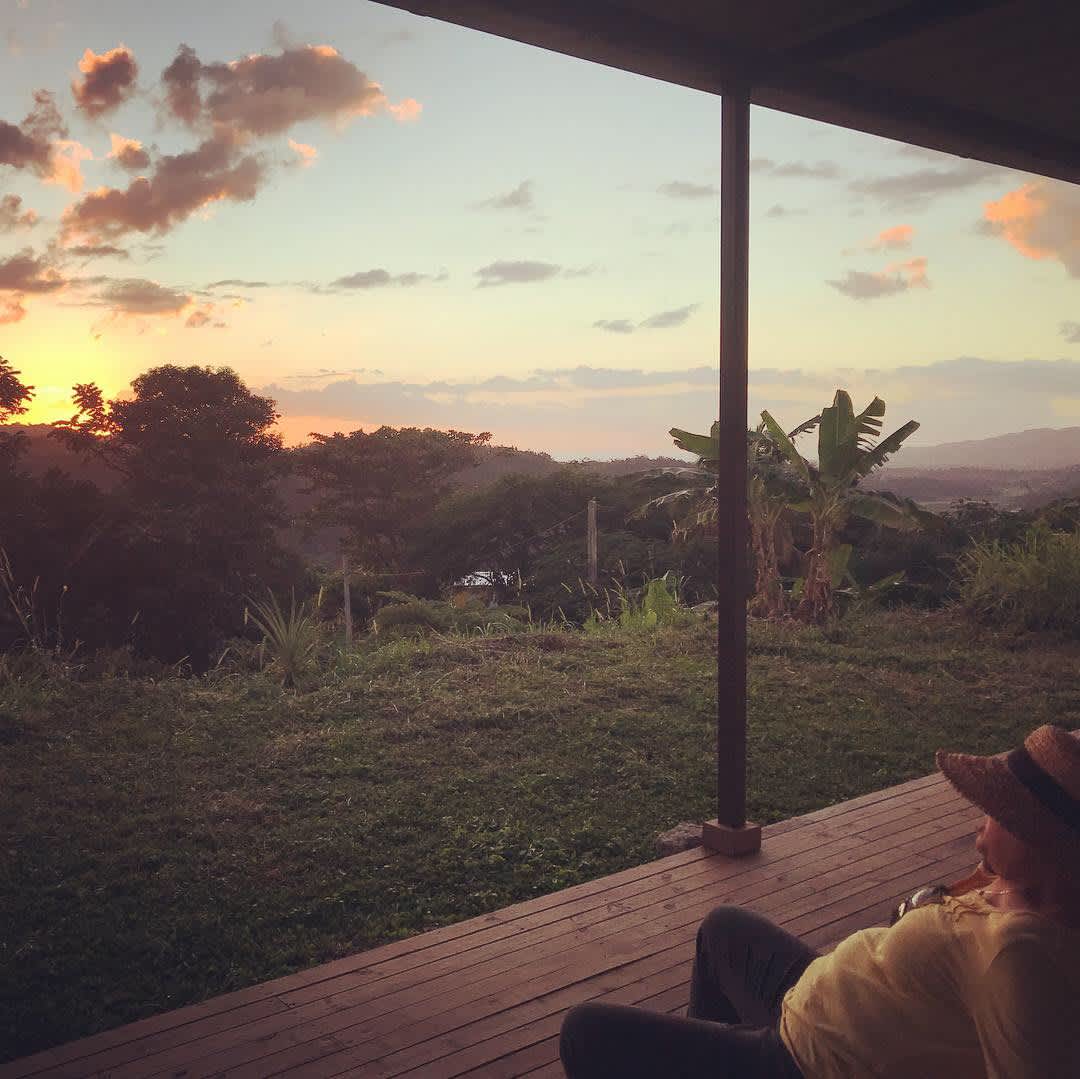In the photograph, a person is sitting on a wooden front porch deck, overlooking a lush, jungle-like landscape as the sun sets. The person, dressed in a yellow shirt, gray or black pants, and a large brown straw hat with a dark brown band, is seated on a chair, absorbing the serene view. The porch has a metal pole supporting the roof, and grass grows in front of the deck. Directly ahead are numerous green bushes and trees, including small palm and banana trees. Off in the distance, there is a house with a silver roof, some hills or mountains to the right, and the sky showcases a vibrant palette of blue, orange, pink, and reddish hues. Wispy gray clouds catch the sun's dying light, amplifying the picturesque scene.